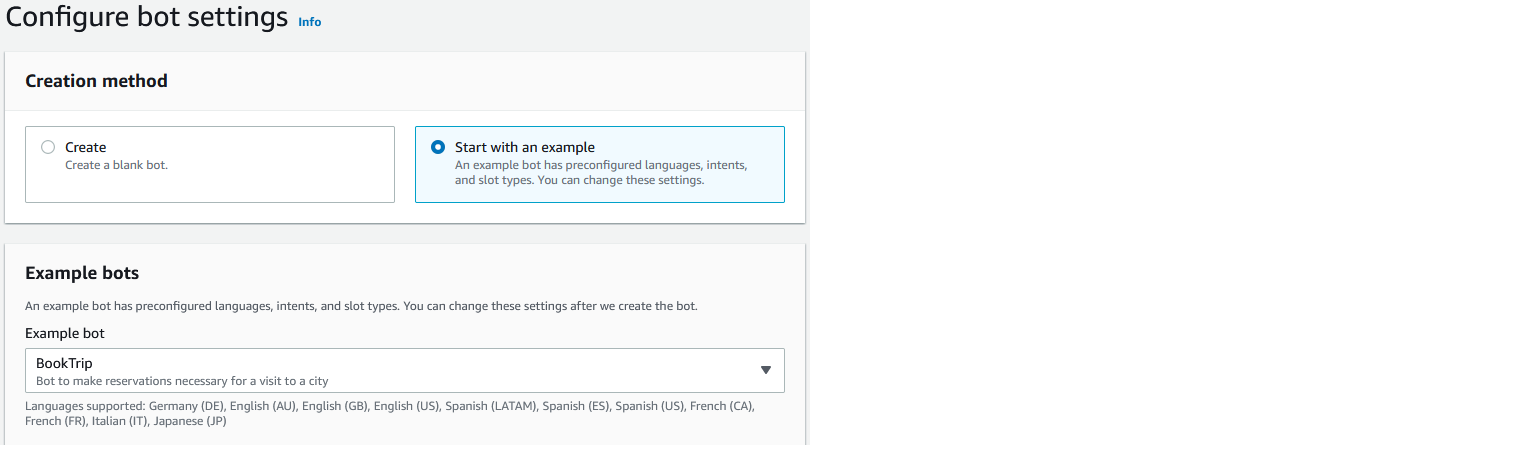The screenshot displays an information page with a gray background dedicated to configuring bot settings. At the top of the page, there is a heading that reads "Configure Bot Settings Info," with the word "info" highlighted in blue. Beneath this heading lies a lighter gray box containing the subheading "Creation Method."

Within the "Creation Method" section, there are two options presented in separate blocks. The first block, labeled "Create a Blank Bot," has a radio button to its left. The second block, labeled "Start with an Example," is highlighted in light blue and selected with a radio button. This option notes that an example bot comes with pre-configured languages, intents, and slot types, which can be modified.

Following this, a section titled "Example Bots" appears in another light gray box, reiterating that example bots come with pre-configured languages, intents, and slot types, which remain adjustable post-creation. Underneath, the subheading "Example Bot" introduces a white box labeled "Book Trip Bot - to make reservations necessary for a visit to a city," accompanied by a dropdown menu to its right.

Below the white box, a list titled "Languages Supported" includes:
- Germany (DE)
- English (AU)
- English (GB)
- English (US)
- Spanish (LATAM)
- Spanish (ES)
- Spanish (US)
- French (CA)
- French (FR)
- Italian (IT)
- Japanese (JP)

The screenshot is partially cut off at this point.